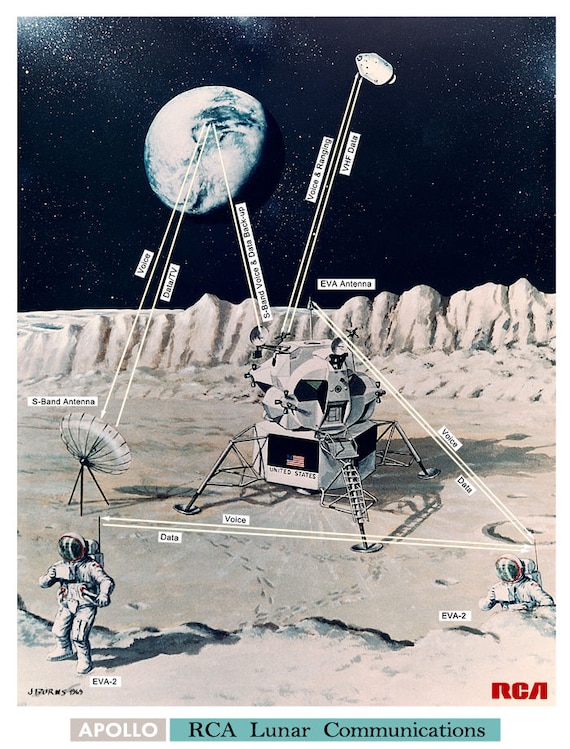The poster is an artistically hand-drawn and hand-colored advertisement for RCA Apollo Lunar Communications, showcasing detailed elements of lunar communication systems. The rectangular poster is bordered by a white frame, with a gray rectangle at the bottom center displaying 'Apollo' in white text, and adjacent to it, a blue rectangle reading 'RCA Lunar Communications' in black text. Above this, the primary image depicts two astronauts on the moon emerging from a crater that houses a lunar lander and a satellite antenna. The illustration, marked with 'RCA' in red text at the bottom right corner, provides a comprehensive diagram of the lunar landing and its communication methods—featuring the S-band antenna pointing towards Earth, indicating voice and data backup channels, and connections to a satellite marked for voice and ranging VHF data. In the background, the moonscape includes a distant cliff and nearby rock formations, with footprints visible in the lunar dust. Communication lines are illustrated from the antennas on the moon lander to the Earth and from the external dish setup to the orbiting mothership, vividly portraying the practical aspects of lunar telecommunications.